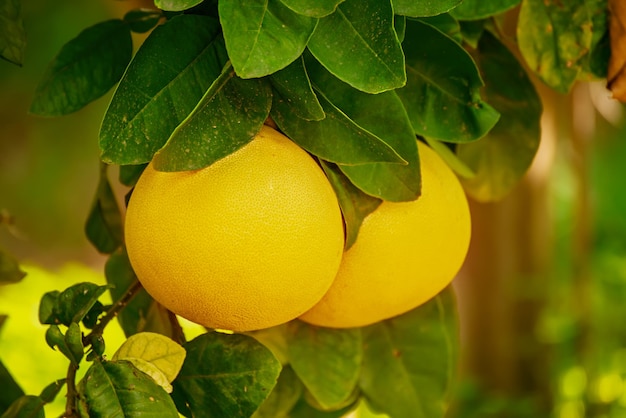This close-up photograph captures two lemons hanging from a branch amidst dense, oval-shaped green leaves with prominent vein patterns. The central focus is on the two bright yellow lemons, with the one on the left being a perfect sphere and slightly in front of the one on the right, which appears a bit oblong and partially obscured by leaves. The lemons' smooth skin features faint dimples. Surrounding greenery and the branch are detailed; however, the background is a blur of various shades of brown and green, drawing all attention to the vibrant lemons in the foreground.